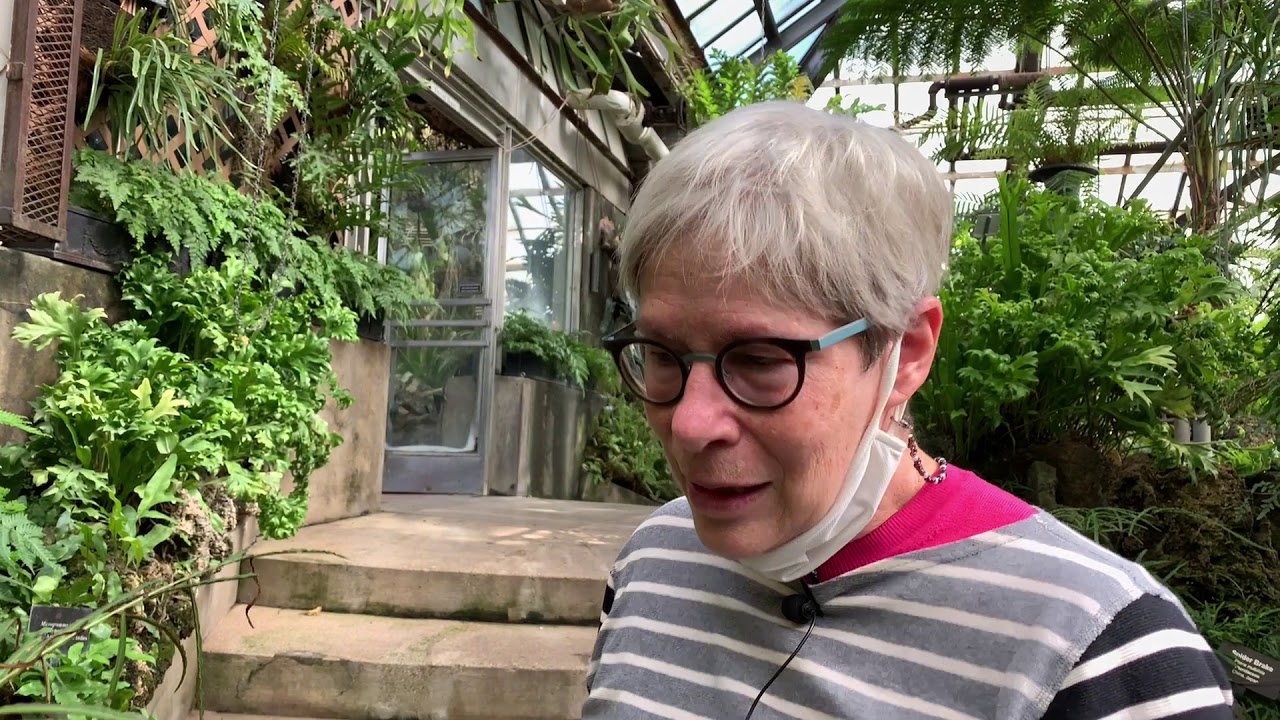The photograph features an elderly woman with short gray hair and distinctive glasses with black lenses and green sides. She wears a face mask pulled down below her chin and has a microphone attached to her gray and white striped sweater, which overlays a pink shirt. The setting appears to be within a greenhouse or botanical garden, as indicated by the glass-covered roof and lush tropical plants surrounding her. To her right, there is a stone staircase leading to a doorway framed with glass doors, which seems to lead to another section of the greenhouse. This additional area appears to be designated for more specialized plant species. The greenhouse is filled with sunlight streaming through the glass roof, creating a warm and inviting atmosphere. The woman stands slightly off-center to the right, looking engaged, possibly speaking into the microphone, suggesting that this image might be a still from a video recording.